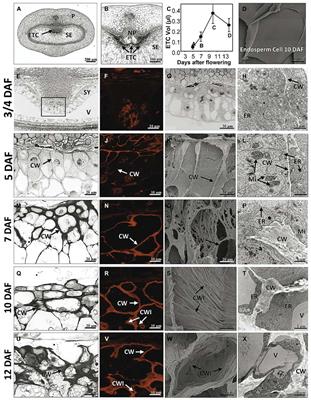This scientific photograph is a detailed collage consisting of 24 smaller images arranged in six rows and four columns. Each image appears to be an up-close, possibly microscopic photograph, with some looking cellular and others potentially geographic, all captured largely in black and white, except for one column which features images with black and red/orange tones.

The columns are labeled A, B, C, and D, with rows marked by the days after flowering (DAF): 3/4 DAF, 5 DAF, 7 DAF, 10 DAF, and 12 DAF. A and B are predominantly black and white microscopic images, while C and D feature small graphs and legends. Each photograph contains indicators or arrows pointing to specific points of interest, marked with labels such as CW, CWI, and TRVX, though their exact meanings are not specified. 

This comprehensive visualization includes a series of legends and axis notations mainly located in the bottom left corners of images, adding to the intricate detailing designed to convey specific scientific information, presumably about a cellular or botanical study.